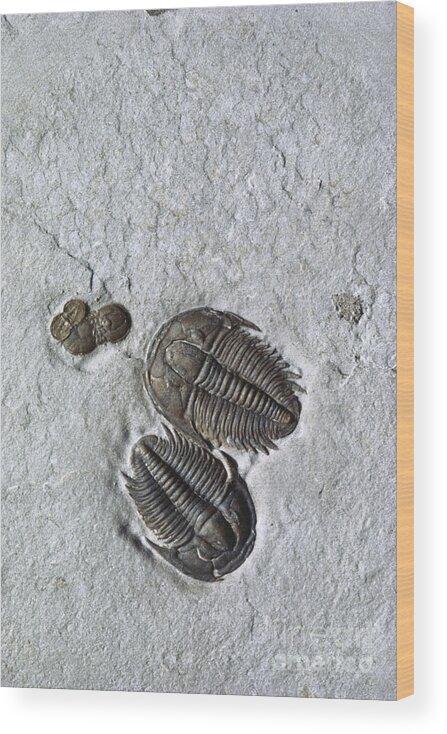The given image features a photograph of what appears to be a fossil embedded in a gray, rocky surface. The central focus is on two large, dark brown, and black fossilized structures resembling ancient, large insects—possibly centipedes or cockroaches—with a smaller, peanut-shaped fossil to the left. The fossil details include a prominent rounded shell or head on one end, followed by multiple legs extending from either side, and a textured, scaly spine with ridges in the middle. Fine cracks run through the gray stone slab, adding to its aged appearance. The background is uniformly gray, and there's a brownish tint on the right side of the image. A white watermark at the bottom reads "Fine Art America." The whole scene is presented in a rectangular block, with the fossils taking up much of the canvas, creating a striking visual element.